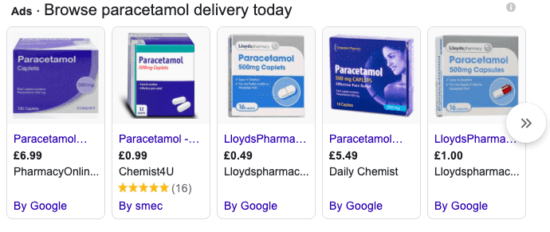This image features a column of advertisements, commonly seen at the bottom of articles on social media platforms like Facebook. At the top, the heading in bold reads: "Ads: Browse Paracetamol Delivery Today." Below the heading, five rows of different paracetamol medications are displayed vertically.

1. **First Row:**
   - **Medication:** Paracetamol
   - **Packaging:** Purple box
   - **Price:** £6.99
   - **Seller:** Pharmacy Online

2. **Second Row:**
   - **Medication:** Paracetamol
   - **Packaging:** Not specified
   - **Price:** 99 pence
   - **Seller:** Chemist For You
   - **Additional Info:** Rated five stars by 16 reviewers

3. **Third Row:**
   - **Medication:** Paracetamol by Lloyd's Pharmacy
   - **Packaging:** White and blue box
   - **Price:** 49 pence
   - **Platform:** Google

4. **Fourth Row:**
   - **Medication:** Paracetamol
   - **Packaging:** Purple box with a woman’s face
   - **Price:** £5.49
   - **Seller:** Daily Chemist

5. **Fifth Row:**
   - **Medication:** Paracetamol
   - **Packaging:** Gray, white, and blue box
   - **Price:** £1
   - **Seller:** Lloyd's Pharmaceuticals on Pharmacy platform
   - **Platform:** Google

To the right of these advertisements, there are arrows suggesting the option to browse additional ads.